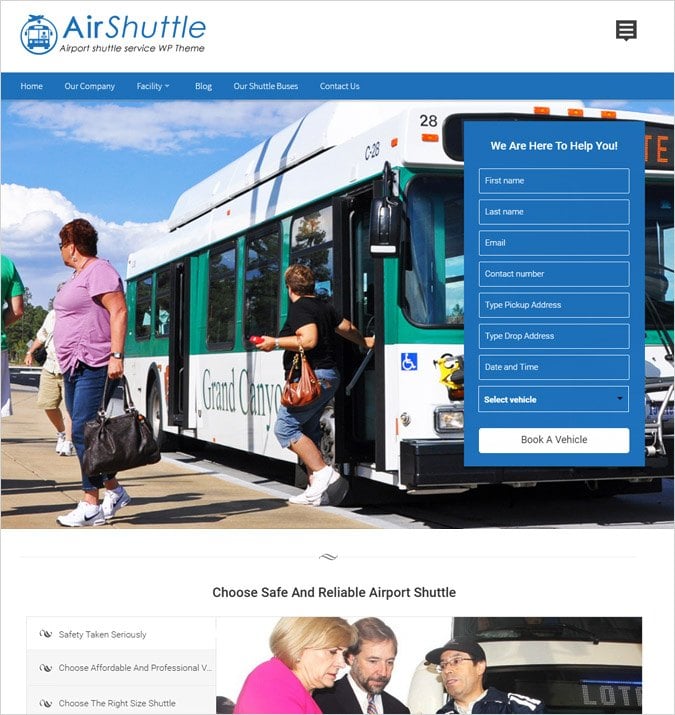**Screenshot of Air Shuttle Website**

At the top left of the webpage, the name of the website, "Air Shuttle," is prominently displayed. The word "Air" is rendered in a dark blue shade, while "Shuttle" is in a lighter, thinner blue. Adjacent to the text logo is a graphic logo depicting a bus heading towards the viewer, colored in the same dark blue as "Air" and encircled by a thin line. Beneath this logo, small black text reads, "Airport Shuttle Service WP Theme."

Directly below the logos, a navigation bar spans across the top left of the webpage, featuring the following options from left to right: Home, Our Company, Facility, Blog, Our Shuttle Buses, and Contact Us.

Dominating the center of the page is a large image showcasing what the shuttle buses look like. The image captures two elderly women disembarking from a bus at a bus stop. One woman, wearing a pink shirt and carrying a brown purse, is walking in one direction, while the other woman, dressed in a black shirt and carrying a black purse, is moving in another direction.

To the right of this central image, text reads, "We Are Here To Help You." Below this slogan is a form that allows users to enter essential information such as their first name, last name, email address, phone number, and both pickup and drop-off addresses, facilitating the planning of their shuttle route.